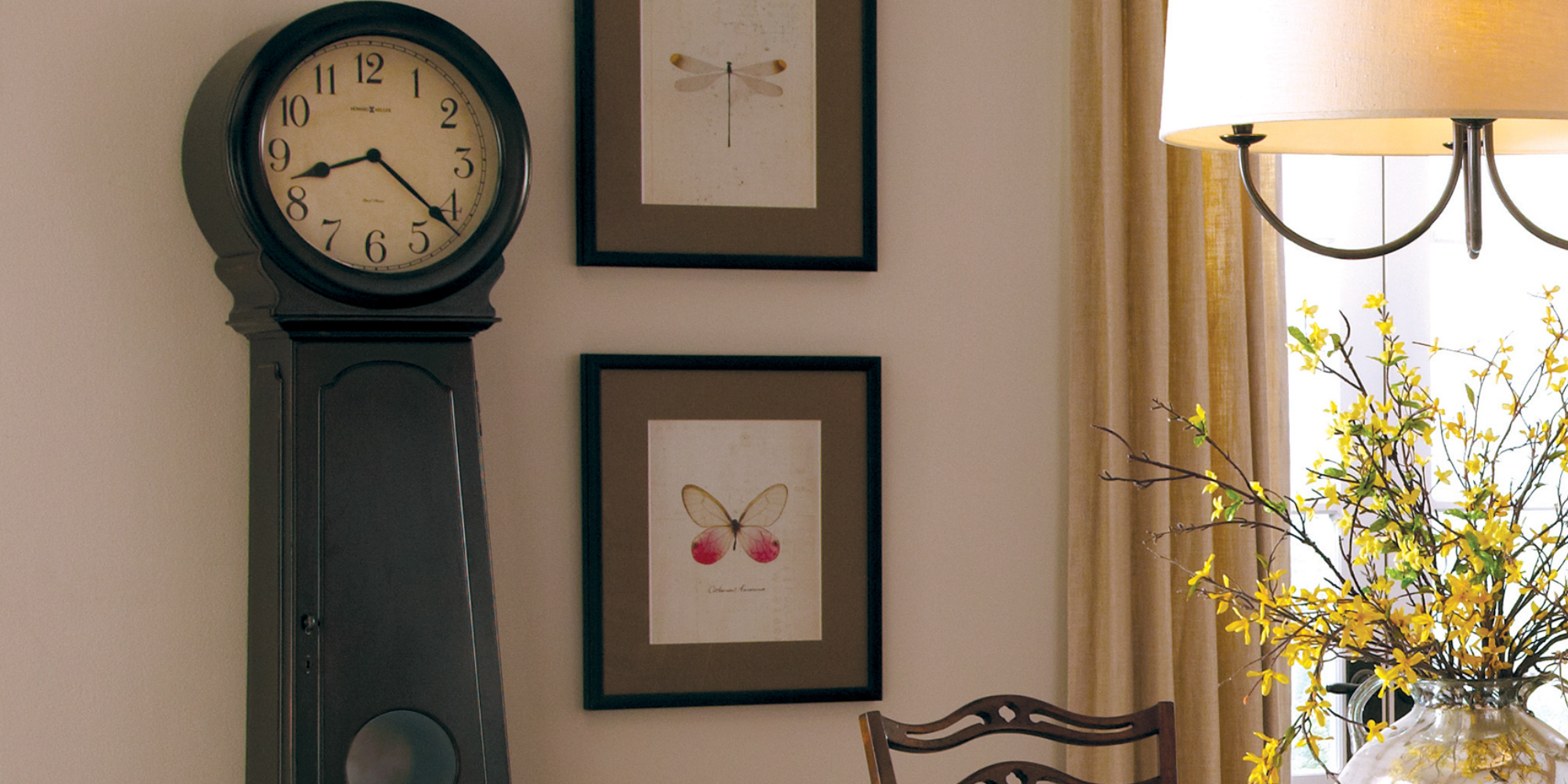In the image, there is a classic black wooden grandfather clock with a tall, tapering base that leads to a round top housing a clock face. The clock face is white with black numerals from 1 to 12 and features black hands indicating the time is between 8:20 and 8:25. The clock is positioned in what seems to be a dining room or living room, up against an off-white wall. To the right of the clock, there are two framed illustrations of insects: a dragonfly at the top and a butterfly below it. A light brown curtain hangs to the right of the illustrations, partially covering a window that lets in bright light. Below the window, there is a table with a clear glass vase containing black stems, tiny yellow flowers, and green leaves. On the left of the vase is the top of a dark brown dining room chair with a wavy design. The room also features a hanging lamp with a shade.